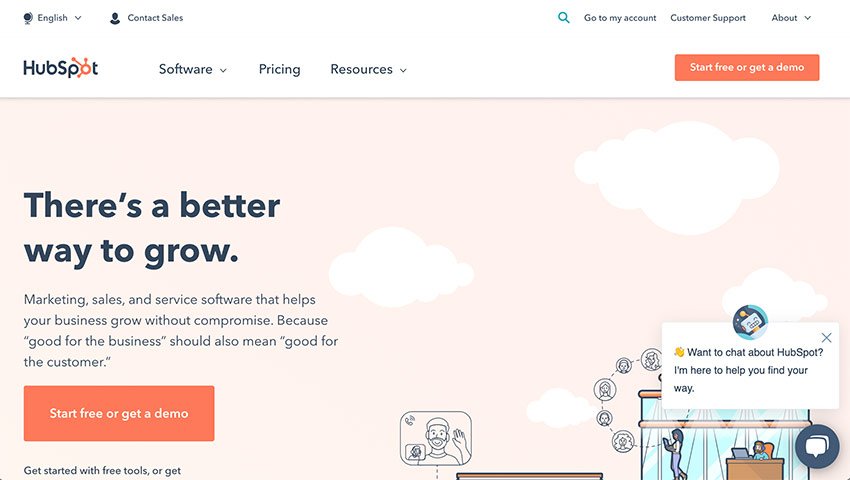Screenshot of HubSpot Website Homepage

This screenshot captures the homepage of the HubSpot website with their branding clearly visible. At the top, navigation options such as "Software," "Pricing," and "Resources" are displayed. The central headline reads, "There's a better way to grow," followed by the subtext, "Marketing, sales, and service software that helps your business grow without compromise. Because good for the business should also mean good for the customer."

Below this main message, there are actionable buttons prompting users to "Start free" or "Get a demo." An additional line starts with "Get started with the free tools or get," but it appears incomplete.

On the side of the screenshot, several icons are visible, emphasizing interactive options like "Start free," "Get a demo," and another icon that prompts clicking. Additionally, there is a chat robot icon accompanied by the text, "I want to chat about HubSpot. I'm here to help you find your way," indicating available customer support.

Website URL: HubSpot.com